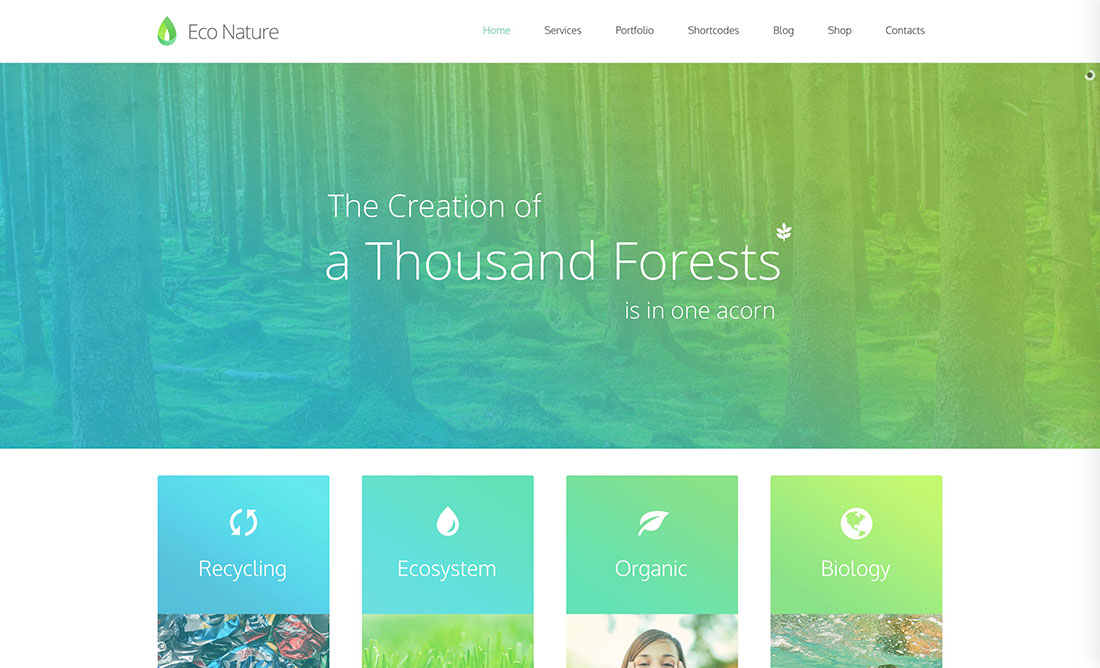This is a detailed screenshot of a website titled *EcoNature*. In the top left corner, there's a green teardrop-shaped logo resembling intertwined ribbons, followed by the text "EcoNature." The navigation menu on the right includes categories in green and black that read: Home, Services, Portfolio, Shortcodes, Blog, Shop, and Contacts. Below the menu, there's a prominent image of a forest, where the left side of the image is tinted blue that gradually fades into green on the right. This forest scene features the text "The Creation of a Thousand Forests and One Acorn" written in white. Just below the forest image, there are four blue boxes labeled Recycling, Ecosystem, Organic, and Biology, each representing different programs or links. The boxes likely contain corresponding images, though these are cropped out of the screenshot.